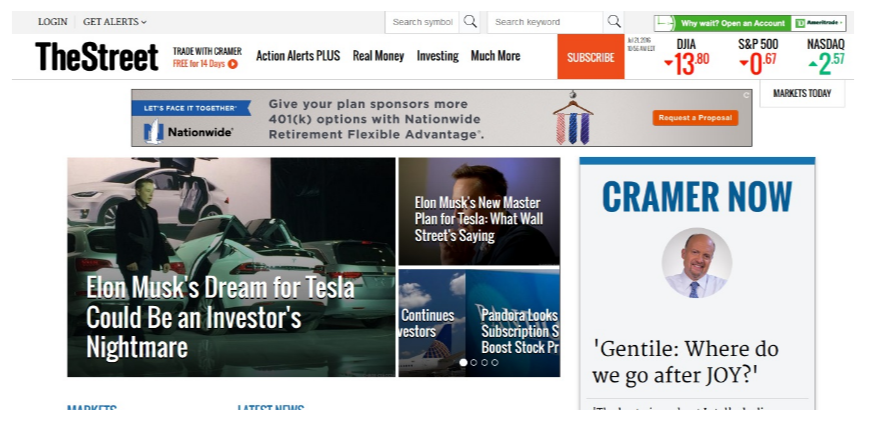This is a screenshot of a Wall Street investing website. At the very top, there is a light gray navigation bar. On the left side of the bar, there are options to log in and get alerts, accompanied by a downward arrow for additional choices. Centrally located is a search bar that offers the options to search by symbol and by keyword. On the right side, there is a small green box with the text "Why wait? Open an account" followed by "Ameritrade."

Further down, a larger box promotes "The Street: Trade with Kramer Free for 14 Days," advertising services such as Action Alerts Plus, Real Money Investing, and more, with a prominent red "Subscribe" button. Below this, current stock information is displayed: the DJIA is down $13.80, the S&P 500 is down $0.67, and the NASDAQ is up $2.57.

A gray box underneath hosts a nationwide advertisement. Below this ad, three article titles are visible: “Elon Musk's dream for Tesla could be an investor's nightmare,” “Elon Musk's new master plan for Tesla: what Wall Street is saying,” and a partially visible title beginning with “Pandora looks,” likely discussing Pandora subscriptions.

On the right side, there is a larger section labeled "Kramer Now," followed by intriguing text: "Genteel where do you, where do we go after joy?"